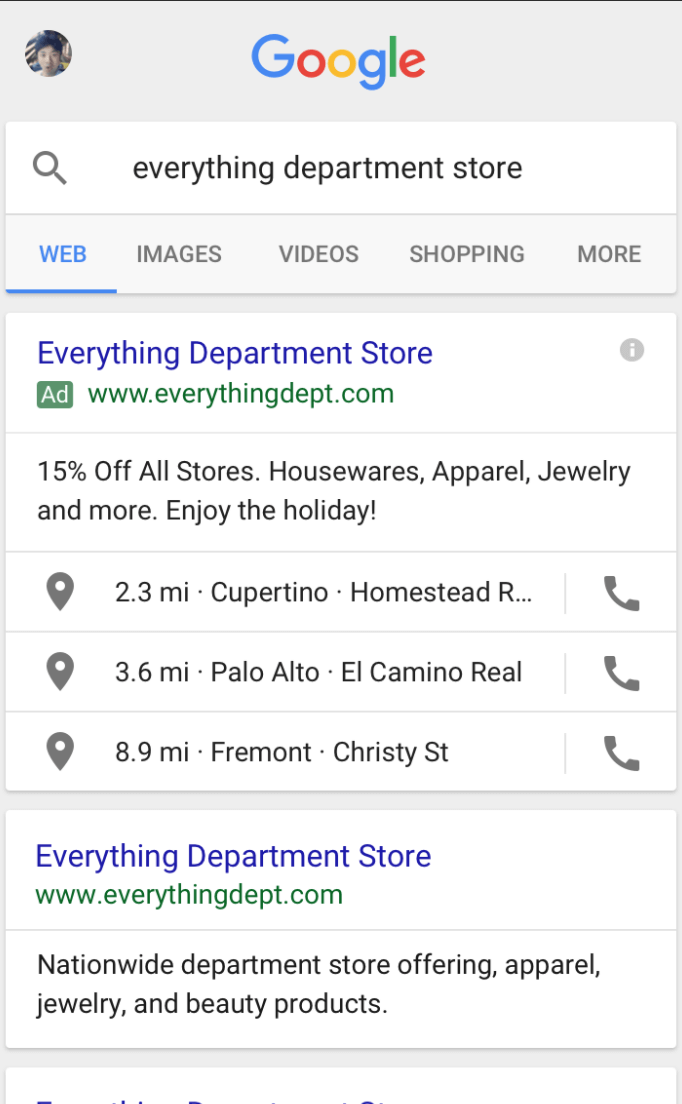A tall, narrow rectangular Google search screen is displayed on a cell phone. At the very top, set in a gray bar, is the distinct word "Google," rendered in its traditional multi-colored letters: the "G" in blue, the first "O" in red, the second "O" in yellow, the second "G" also in blue, the "L" in green, and the "E" in red. Adjacent to the Google logo is a small, circular thumbnail image featuring a black-and-white photograph of a young man.

Beneath this, a white search bar is prominently positioned, displaying black text and a small magnifying glass icon. The phrase "everything department store" has been entered into the search bar, and a search has been executed.

Directly below the search bar are tabs for different search categories: "Web," "Images," "Videos," "Shopping," and a general "More" category. The top search result is a link to the Everything Department Store website, indicated as an ad from everythingdepartment.com. Additionally, it provides details on the store's location relative to the user.